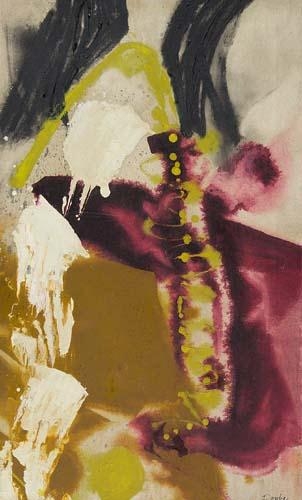This abstract painting features a composition of deep and contrasting colors including burgundy, maroon tinged with purple, mustard yellow, ochre, black, gray, and white. The background is predominantly gray with striking black brushstrokes descending from the top. Between these black markings, there's a distinct yellow shape resembling an upside-down "V." Alongside, white splotches spread across various parts of the artwork, notably clustered on the left and at the bottom where they are juxtaposed with three large red splotches. The mustard yellow forms a dynamic element with dots and streaks that traverse the center, while a deep burgundy or reddish-violet hue dominates significant areas, especially on the right, accented by yellow spots. The composition is highly experimental and abstract, with no discernible objects or text, although some paint blotches evoke the semblance of unreadable letters. The deliberate randomness and bold, vivid colors create a visually arresting and unresolved piece.